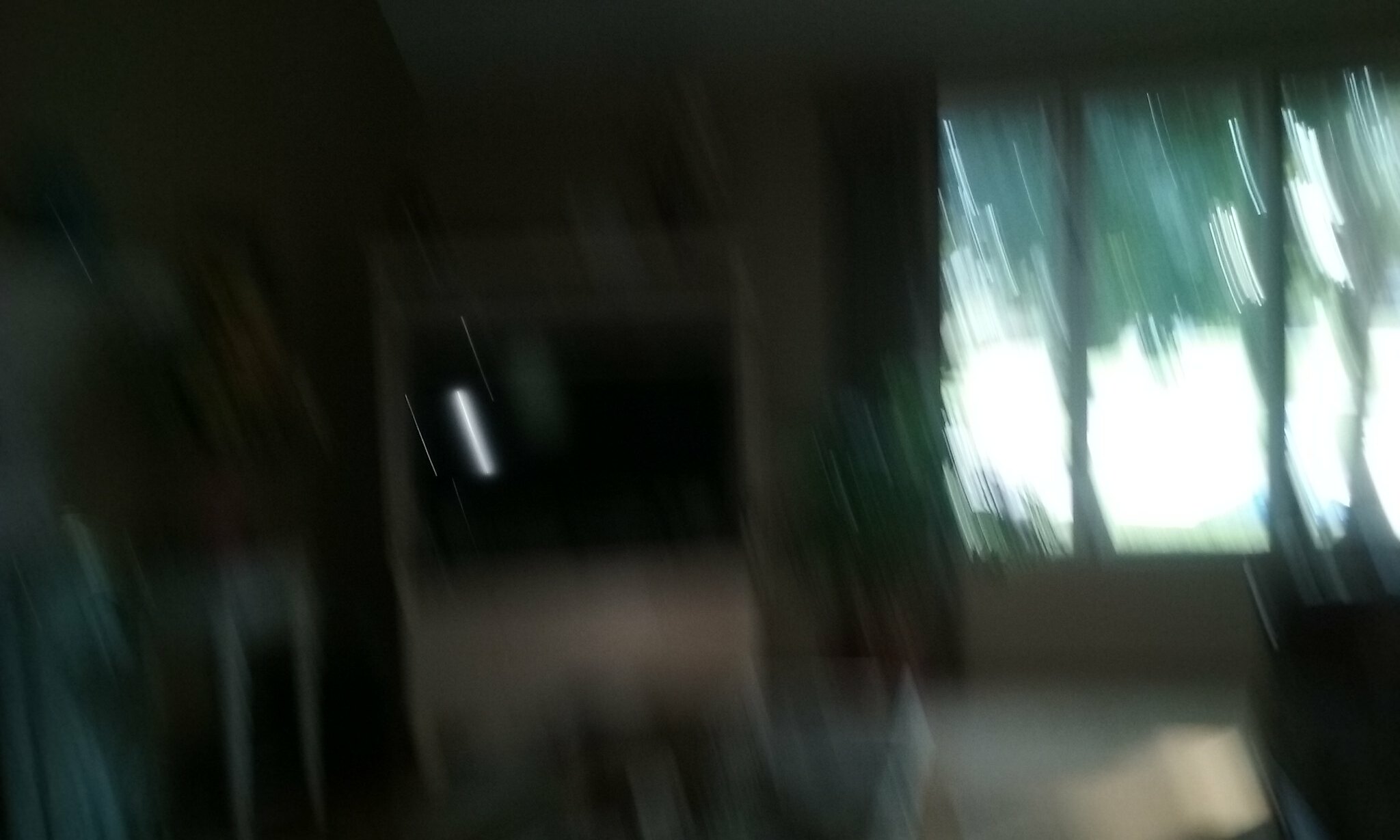This color photograph is extremely dark and blurry, making it difficult to discern precise details. The image appears to depict a dimly lit room within a house. At the center, there is a dark, indistinguishable object that seems to be a TV set, which is currently turned off. To the left, a white table is faintly visible. On the right side of the photograph, a window with the curtains drawn open allows a soft light to spill into the room. The top section of the image shows a dark green, blurred area that could either be trees outside the window or possibly curtains. The photograph, wider than it is tall, lacks any textual elements. The overall blurriness and darkness render many elements of the scene unclear, contributing to its indistinct, enigmatic quality.